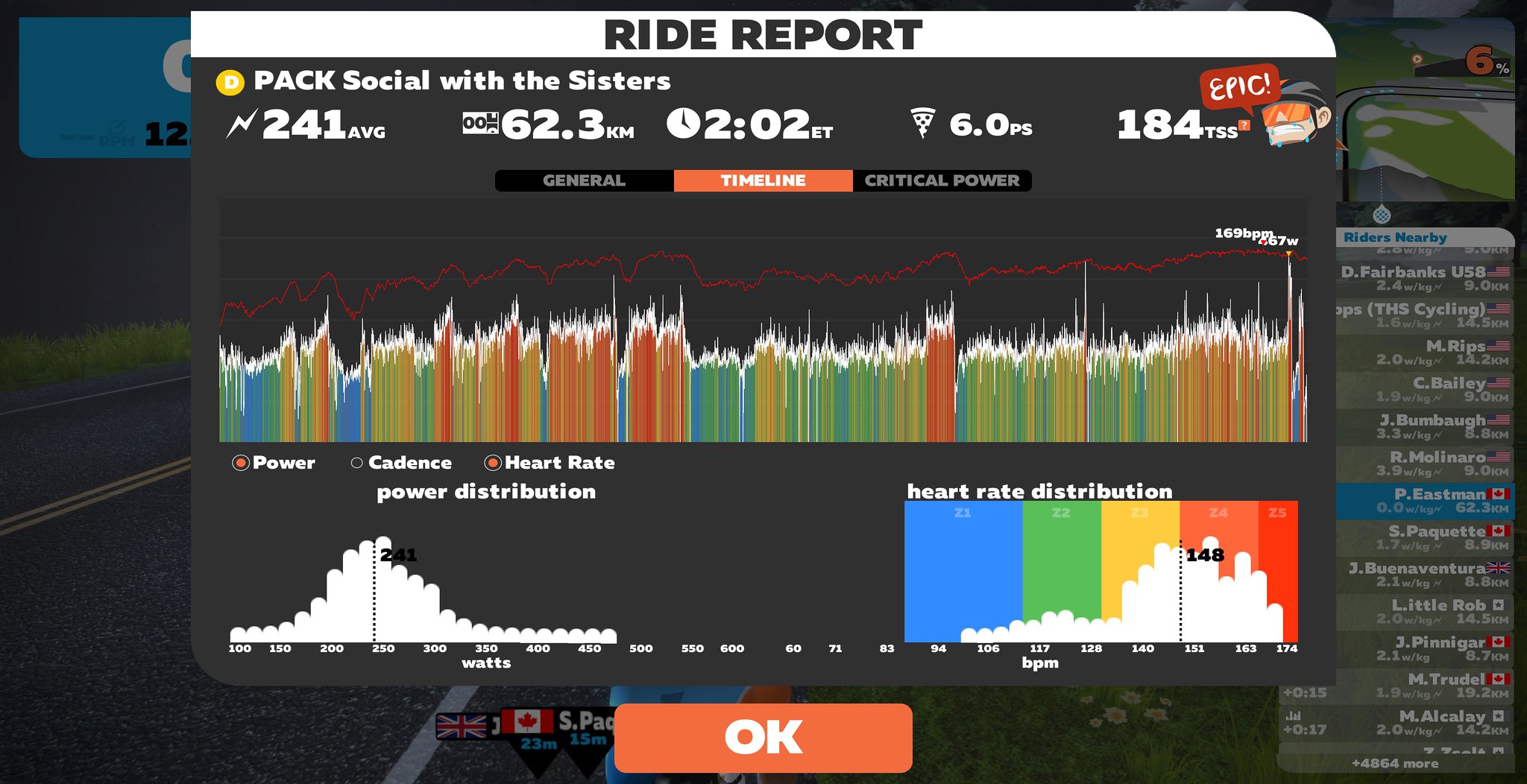This detailed image depicts a Ride Report screen commonly associated with a Peloton or another high-tech exercise bike. At the top, set against a white background with bold black text, it reads "Ride Report." Directly below, in white text against a black background, it says "Pack Social with the Sisters." The upper left corner displays "241 AVG," presumably indicating the average power output, while to the right, it lists "62.3 kilometers" and the time "2:02 Eastern Time." Further to the right, it reads "6.0 PS" and "184 TSS" with a small red banner above it labeled "Epic."

Underneath these metrics, the screen features a colorful, dynamic line graph showing power output with varying hues of blue, orange, and white. Below this graph, labeled in small white text, are categories for "Power," "Cadence," and "Heart Rate." Following this, there is a graph illustrating power distribution starting at 100 watts and peaking at 283 watts, tapering down to 400 watts at the lower right.

Adjacent to the power distribution chart is a heart rate distribution graph, which showcases four columns in blue, green, yellow, and red. The activity level begins low in blue, escalates through green and yellow, and peaks in red before declining.

At the bottom of the screen, an orange banner displays a prominent "OK" in white letters. To the right, a vertical list of names, likely representing riders or organizations who have used the meter, is faintly visible. This vibrant and data-rich screen provides users with detailed performance metrics, enhancing their workout experience.